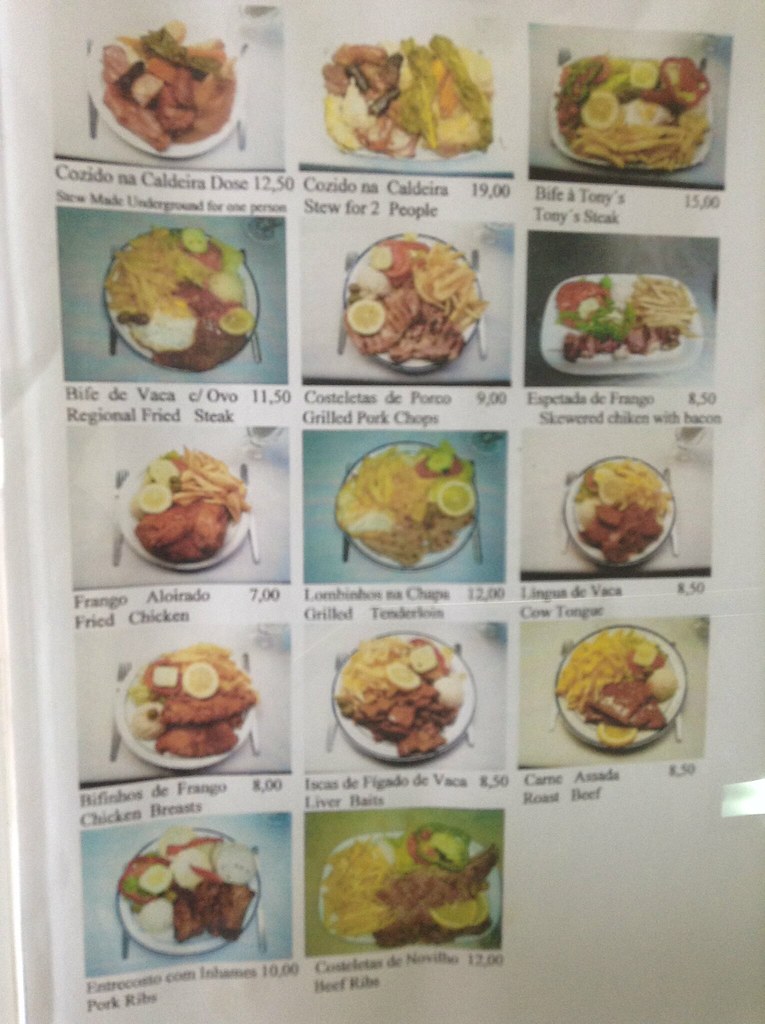The image features a Spanish-language menu divided into three rows, each showcasing various dishes. The menu includes multiple photographs of meals, though the images are quite blurry. Each photo prominently displays a meat item, with some accompanied by corn. Notably, no dishes seem to contain any green vegetables. Several items are served with a generous portion of fries. Prices for all the menu items are relatively low. Interestingly, the last row of the menu does not include a third photo, leaving a space.